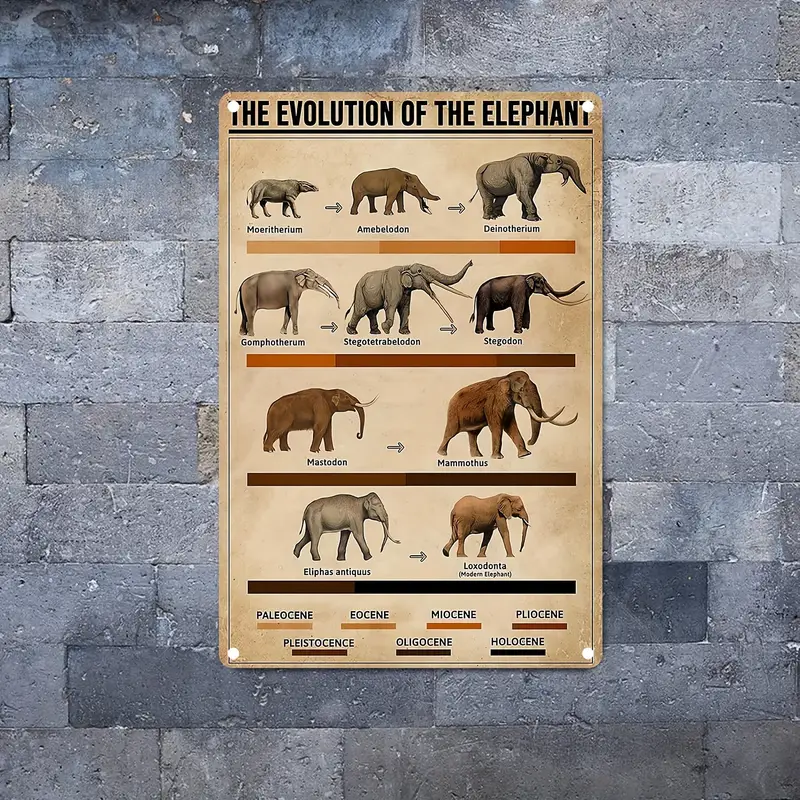The image showcases a detailed chart titled "THE EVOLUTION OF THE ELEPHANT" in black, uppercase letters at the top, affixed to a gray, gradient-shaded cinderblock wall with four white dots implying attachment at the corners. The poster resembles an antique document, with its background transitioning from tan to darker shades of brown. It features ten distinct stages of elephant evolution, organized into four rows of images: three stages on the first row, three on the second, two on the third, and two on the fourth. Each row is separated by progressively darker bars, visually marking different geological time periods. The chart includes scientific labels beneath each image, representing various time periods such as Paleocene, Eocene, Miocene, and Pliocene, among others. The background colors on the chart vary, incorporating hues of gray, brown, white, red, and black, which enhance its historical and educational appeal.